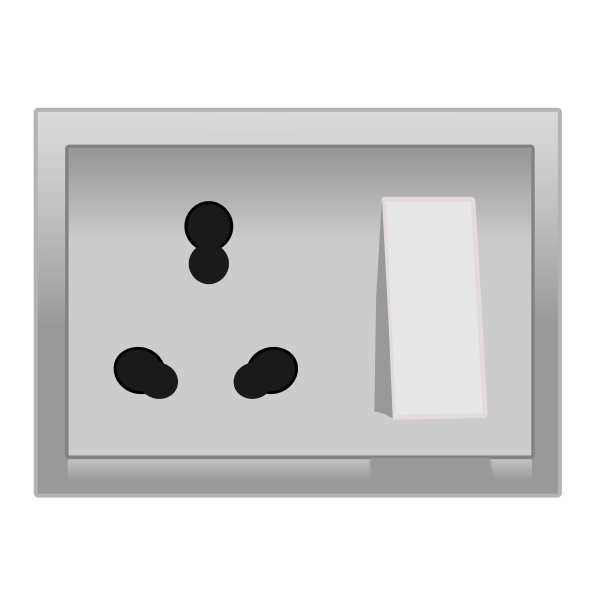The image is an abstract, computer-rendered graphic art piece presented within a light gray frame, which resembles either a screen or a picture frame. Inside this frame, the background transitions from a darker gray at the top to a lighter gray at the bottom, framed by a gradually darkening outer border. On the left side of the image, there are three black circular shapes, reminiscent of footprints, push pins, or clumped circles, arranged in a triangle – one on the left, one on the right, and one on top in the middle, with some overlapping elements. On the right side, there is a tall, narrow, off-white rectangular structure that resembles a door or a wedge-like object, casting a dark gray shadow on its left side. The overall style of the graphic is non-realistic, leaning towards clip art with an abstract feel.